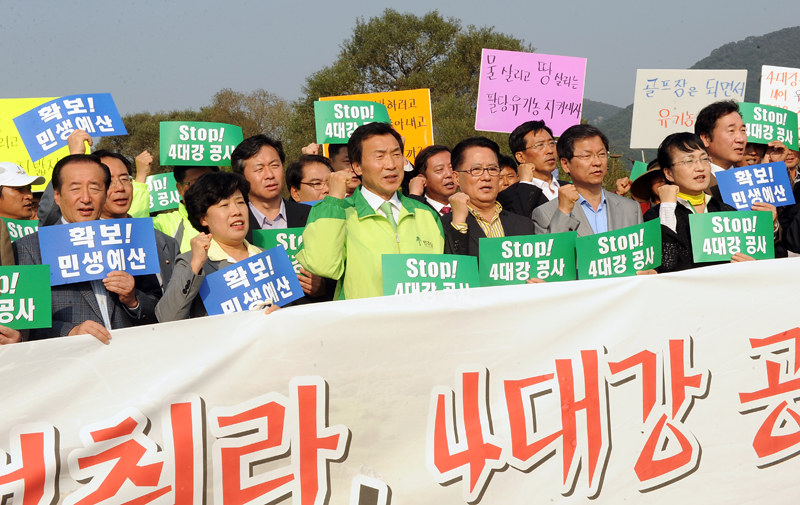In the photograph, a crowd of predominantly older Asian individuals is gathered, engaging in what appears to be a protest. Dominating the foreground is a large white banner with red Asian or Japanese characters, occupying about half of the image. The protesters are also holding an array of multicolored signs, with many reading "STOP" in white lettering on green signs, underlined by Korean characters. Blue signs and various hand-drawn ones also feature Korean text. Most people in the crowd are wearing jackets and suits, with several participants raising one fist in the air. The setting appears to be outdoors during the day, with a background that includes mountainous regions on the right and trees with bright green leaves partially obscuring the sky, which is a grayish hue. The crowd and the signs they are brandishing are centrally positioned in the photograph, indicating a well-organized demonstration.